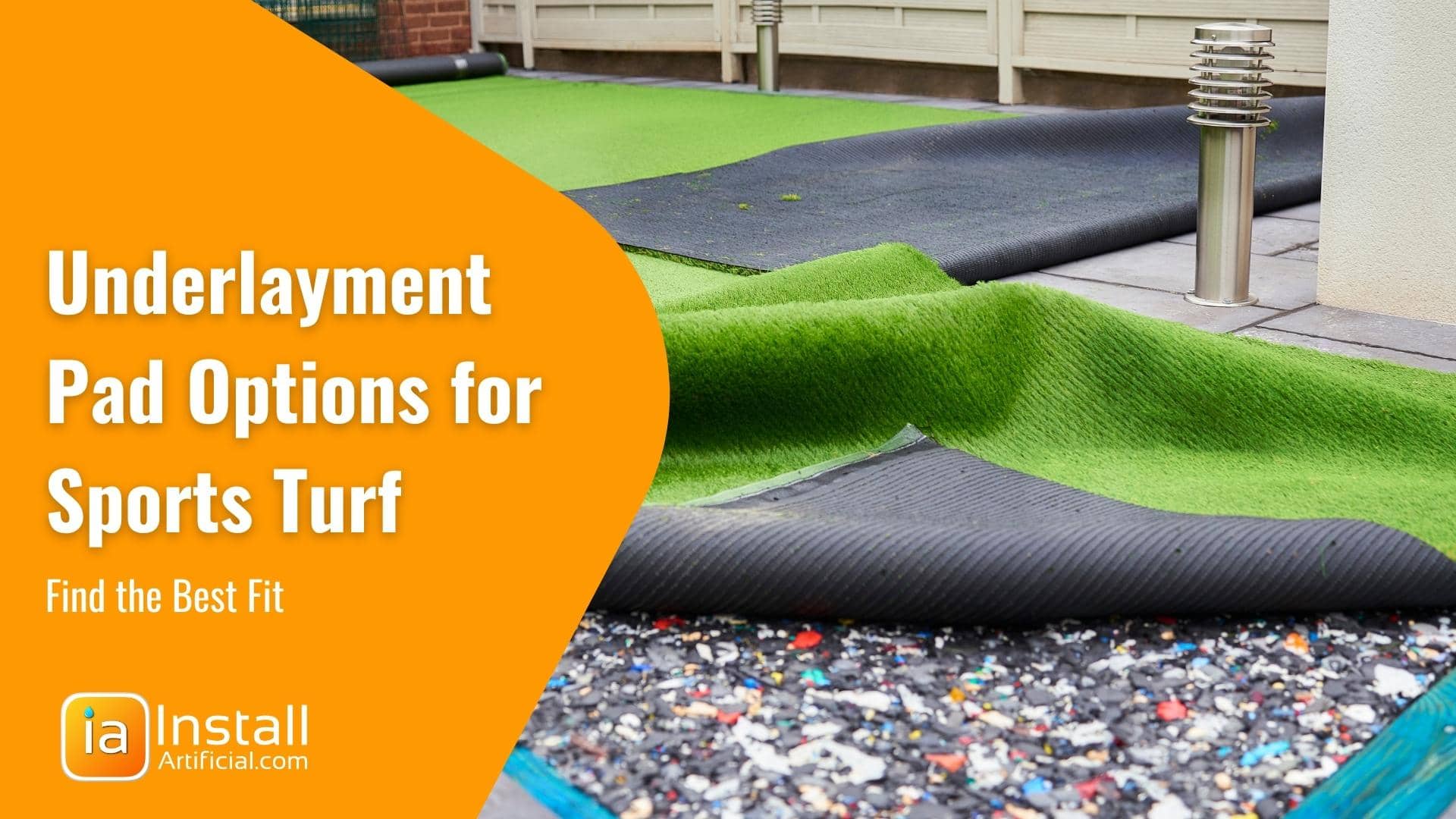This image is an advertisement showcasing options for underlayment pads used beneath artificial sports turf. The picture features two patches of green synthetic turf, often seen in sports arenas, partially peeled back to reveal colorful and seemingly springy underlayment, which appears to be made of recycled compressed rubber. Dominating the left side is a large orange banner with white text that reads, "Underlayment Pad Options for Sports Turf. Find the Best Fit." Beside this banner, the logo "ia" with a turquoise dot over the "i" appears, along with the website "installartificial.com" in smaller text. This informative visual highlights the padding solutions designed to offer protection and comfort during sporting activities, ensuring a safer and more enjoyable experience on artificial surfaces.